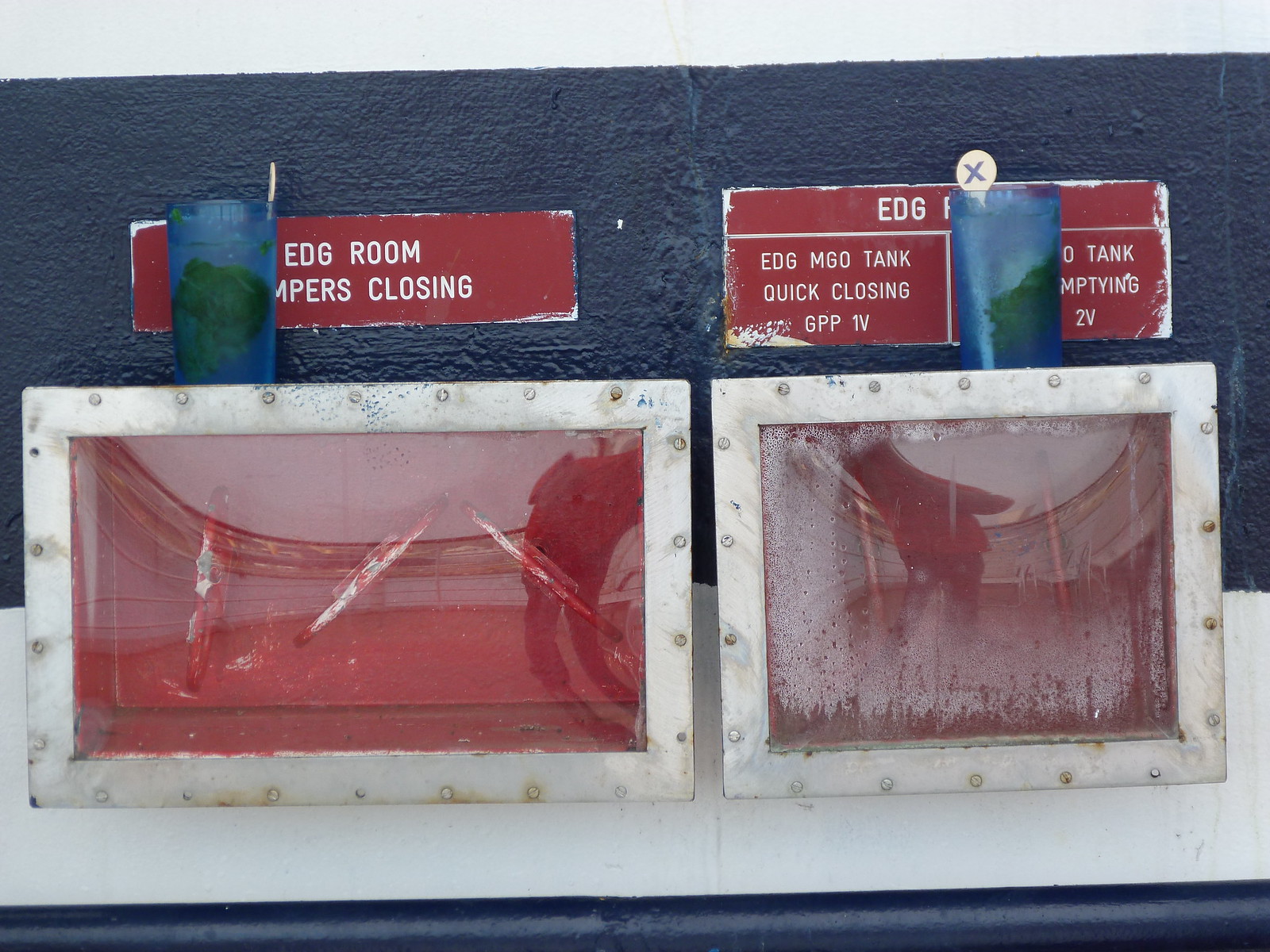This photograph depicts two metal-framed chambers, side-by-side, set on a stark white countertop against a dark blue wall. The left chamber is rectangular, while the right chamber is square, each containing a smearing red liquid, which could either be paint or blood. Both frames are silver with visible bolts, giving them a rugged, industrial appearance. The condensation clinging to the insides of the clear plexiglass emphasizes the mysterious and possibly scientific nature of the setup.

Above each chamber, there are partially obscured red labels with white, sans-serif text, likely made of metal. The label over the left rectangular chamber reads: "EDG room M-P-E-R-S closing," with some letters cut off by the adjacent blue objects. The label above the square chamber reads: "EDG MGO tank, quick closing GPP 1V, tank emptying 2V."

Adding an element of intrigue, blue plastic cups with water and green leaves are placed atop the steel frames, partially blocking the view of the signs. The entire image exudes a sense of scientific experimentation or industrial process, enhanced by the deep, contrasting colors—burgundy red, dark blue, gray, silver, black, and white.